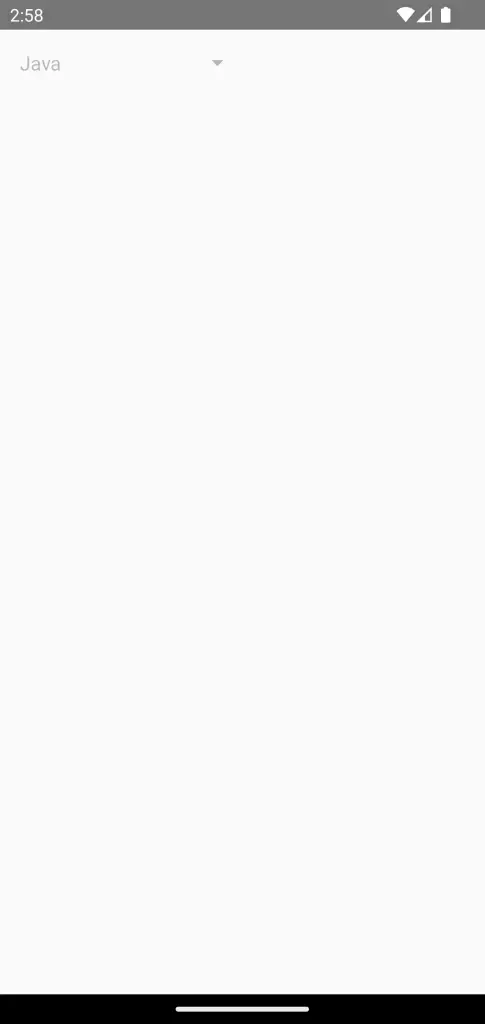The image appears to be a screenshot from a mobile device, displayed in portrait orientation. The top portion of the screen features a dark gray bar, which includes several elements: on the left, it displays the time "2:58"; on the right, it showcases three white icons representing Wi-Fi connectivity, signal strength, and battery status.

Below this dark gray bar, the majority of the screen is filled with a lighter gray background. Positioned centrally on this lighter backdrop is a single menu option labeled "Java" in light gray text. Adjacent to this label is a small triangle icon, indicating a drop-down menu, though it appears to be minimized, with no options listed beneath it.

The overall layout is rectangular and significantly taller than it is wide. At the very bottom of the screen, there is a black border containing a thin white line, which forms the concluding part of the image.